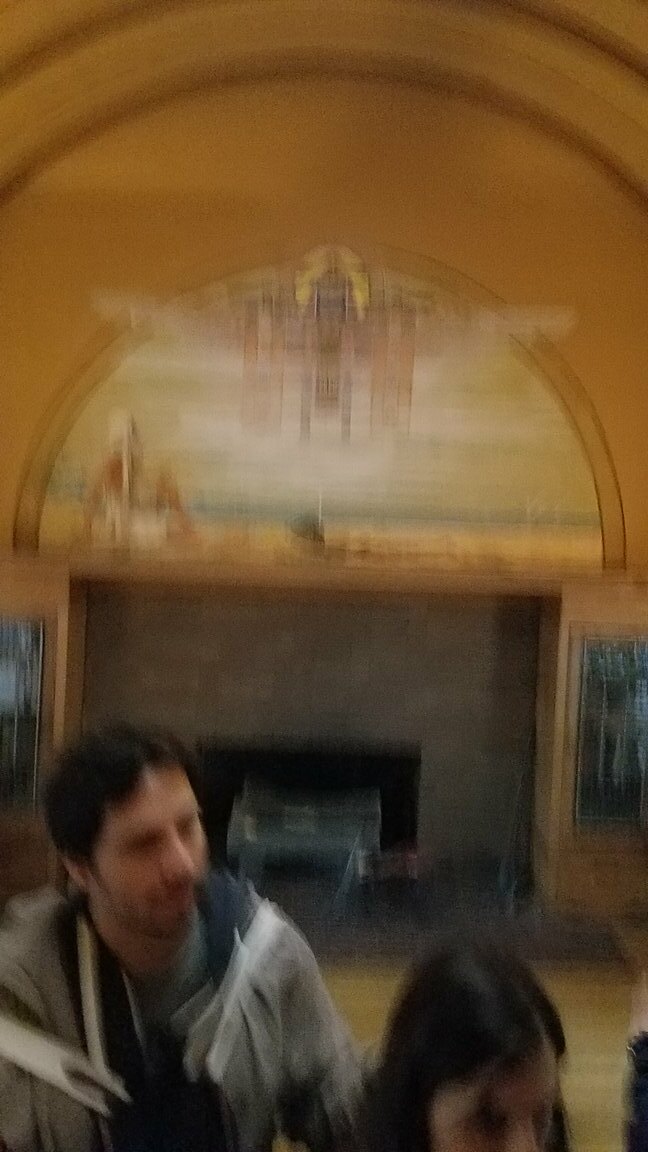The image is a blurry, color photograph taken in narrow portrait mode, depicting an indoor setting that resembles either a museum or a church. In the foreground, there are two people. On the left is a young man with dark hair and a beard, wearing a gray jacket over a blue hoodie. He appears to be looking down towards the right. Next to him, on the right, is a woman whose head is partially cropped and whose gender is determined by having long hair. Both individuals are very blurry.

In the background, there is a large stone fireplace surrounded by brown bricks. Above the fireplace, there is an arched ceiling featuring a semi-circular painting that potentially includes religious figures, indicated by the attire of the people in the artwork. Despite the blurriness, hints of stained glass windows can be seen on the sides. There might also be a cutout area behind the figures that possibly houses a piano, and a guitar stand is visible on the right side. The photo does not contain any legible writing, animals, or plants.